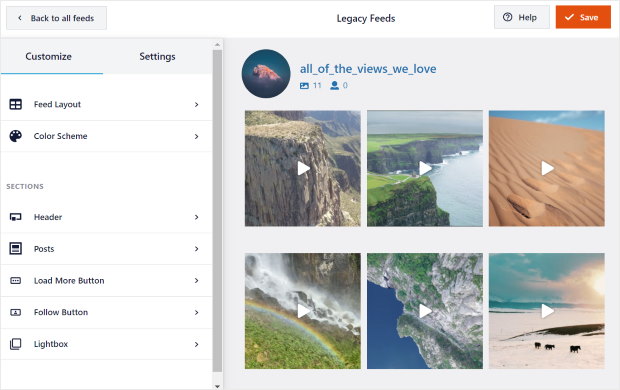The top left corner of the image features a grey section with the text "Back to All Feeds" and "Legacy Feeds." Nearby, there is a grey square labeled "Help" and buttons for "Save," "Access Customize Settings," "Feed Layout," "Color Scheme," "Instructions," "Header," "Pause," "Load More," and "Follow." 

On the very right is another grey square adjacent to a set of photos. The section titled "All of the Views We Love" includes 11 photos. The collection captures various natural landscapes: a mountain range, two bodies of water, green hills, desert dunes, a blue sky with a rainbow, more water scenes, mountains, grassy fields, rocky terrain, and a bright sun. One photo shows a desert scene with three animals walking across it. The image is bordered by grey lines and includes another "Load More" button, a "Follow" button, and a lightbox feature for photo viewing.